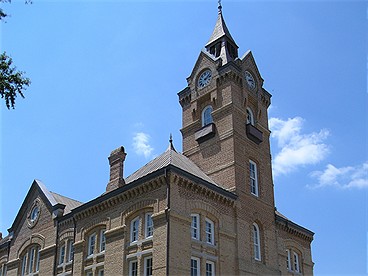The photograph depicts a grand, brown brick building or castle, wider than it is tall, with a large pointy tower on its right side. Captured from a low angle, the image presents a clear blue sky with a few light clouds in the background. Some tree leaves hang down from the top left corner, adding a natural touch to the scene. The tower on the right side of the building extends several stories above the main structure, which is visible up to two stories high. The majestic structure features long, curved white-framed windows that reflect the sky. There's a triangular top on the left side with a circular window. The imposing tower has clocks on at least two of its four sides and ends in a triangular point with a circular detail at the top. The building gives an aura of an expensive manor or perhaps a cathedral or university, with its elaborate architecture highlighted against the serene sky. No people are visible in the image, which emphasizes the grandeur and solitude of the scene.